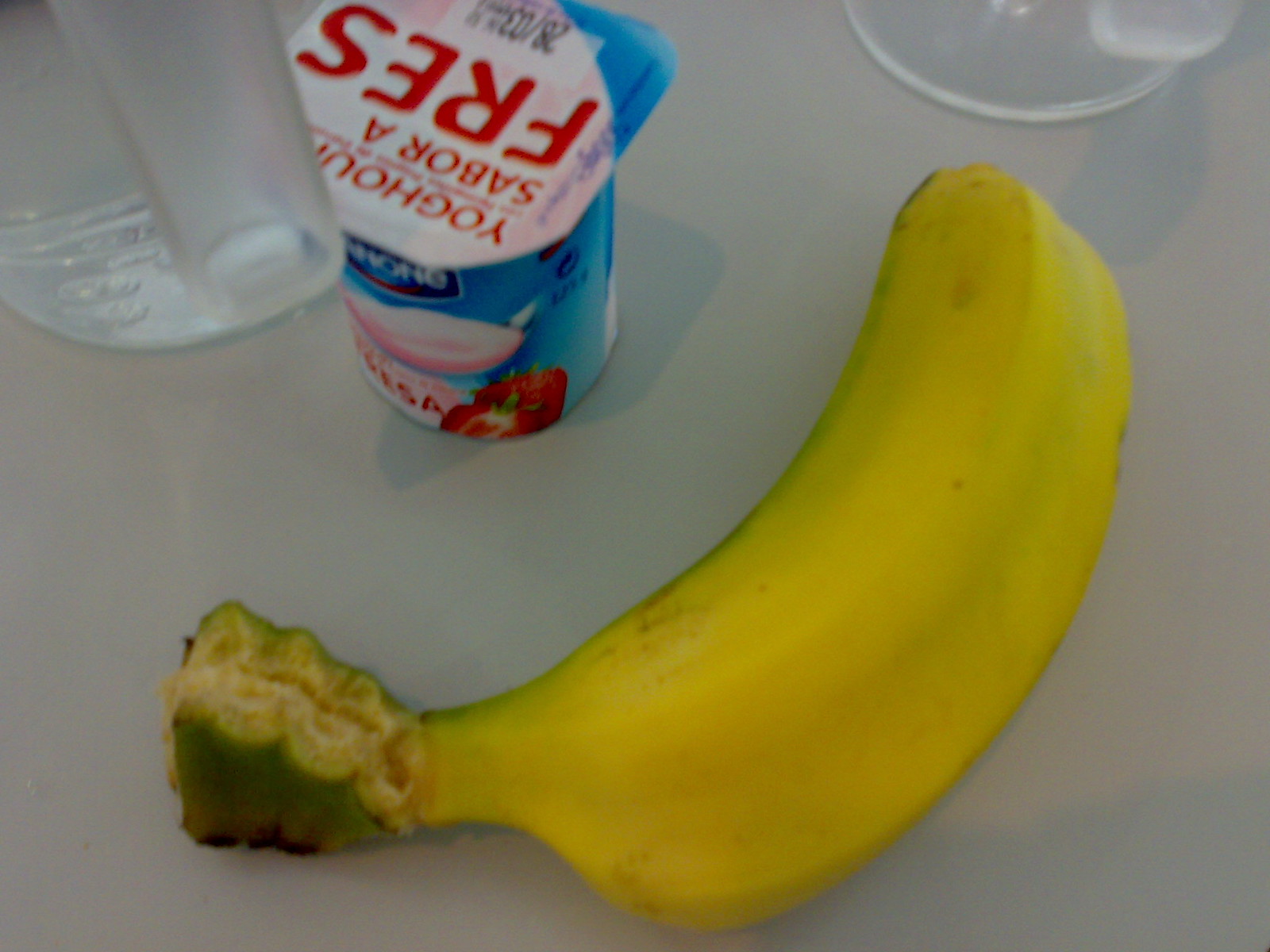In the photo, slightly out of focus, lies a small banana on a white table. The banana, still attached to its greenish stem, shows signs of having been part of a trio until recently. The stem, along with part of the banana's peel, retains a touch of green while the majority of the peel is yellow. The banana is positioned such that the stem and the tip rest at the bottom left corner of the image, curving upward toward the top. 

Next to the banana is a Dannon yogurt container. The top label of the yogurt is blue, featuring the Dannon logo, along with the word "yogurt" in Spanish ("sabor A FRES"). The label is adorned with a picture of a pink spoonful of yogurt and a couple of sliced strawberries. Adjacent to the yogurt is a clear plastic container, partially visible. Additionally, a clear, circular base of what appears to be a glass is located next to the banana, near the yogurt container.